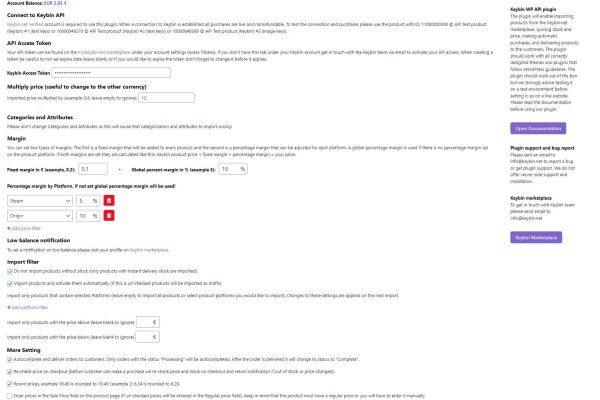This is a detailed description of a cluttered and largely unreadable screenshot from an unspecified source. The top of the image shows the text "account balance," followed by an unintelligible word, and then "API." Below it, smaller indistinguishable text precedes "API access token" followed again by blurry writing, then "account access token." Further down, terms such as "multiply price," "useful to change to the other currency," "categories and attributes," "margin," "percent margin by platform," and "low balance notification" are faintly visible. Additional sections include "import filter," "more settings," a vertical area to the right mentioning "API plug-in," "plug-in support," and an unclear term before "report," along with a reference to something related to a marketplace. The image does not include any photographic elements, people, animals, plants, automobiles, motorcycles, or bicycles, and it is entirely composed of textual content that is largely too small and blurry to be legible.